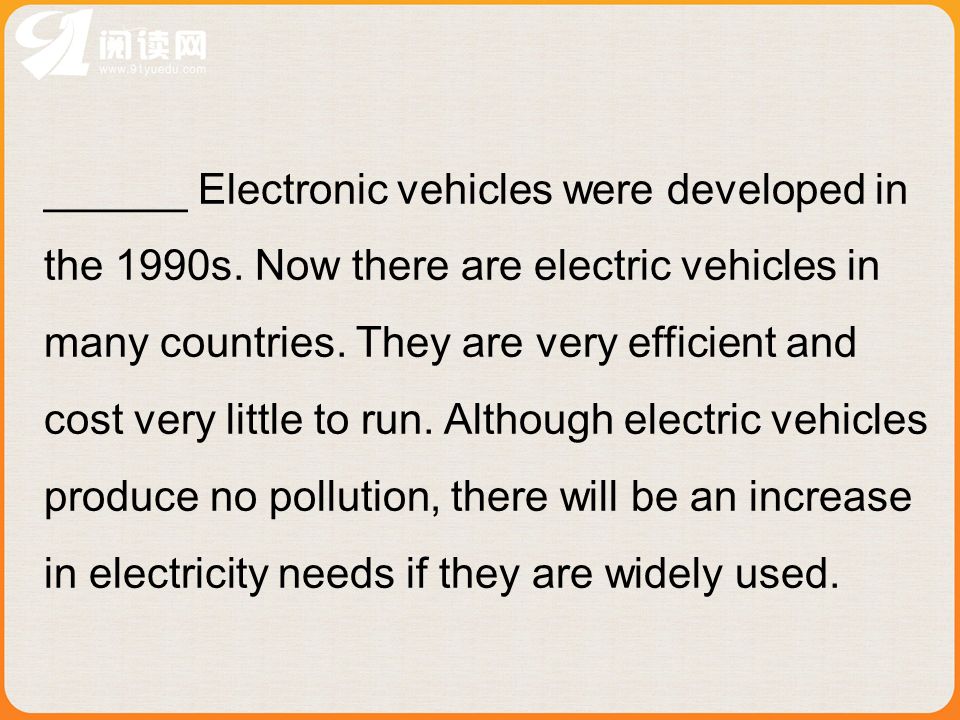The image displays a rectangular text box with a light gray, beige-toned background and a thin orange border that thickens at the corners. Dominating the center of the box is a block of black text in a sans-serif font. The text reads: "Electronic vehicles were developed in the 1990s. Now there are electric vehicles in many countries. They are very efficient and cost very little to run. Although electric vehicles produce no pollution, there will be an increase in electricity needs if they are widely used." In the upper left-hand corner, there is a white logo featuring a stylized crescent moon shape possibly incorporating the number one and what appears to be a cape, accompanied by some Asian characters, likely Chinese, underneath it. The website www.91yuedu.com appears below the logo.